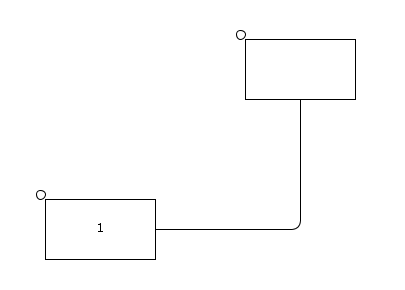This digital image appears to be a computer-generated graphic, possibly designed as a set of instructions or a schematic showing connections between components. The graphic features two outlined rectangles, each with a small outlined circle located at the top left corner outside the rectangle.

The rectangles are positioned diagonally from one another, with the top rectangle situated higher and to the right of the bottom rectangle. Extending from the center of the top rectangle is a line that travels downward almost to the bottom of the image. Upon reaching the lower part of the graphic, the line makes an L-shaped turn to the left, eventually connecting to the bottom rectangle. Inside the bottom rectangle, the number "1" is prominently displayed. This detailed arrangement likely serves to illustrate a particular flow or connection between the two components represented by the rectangles.